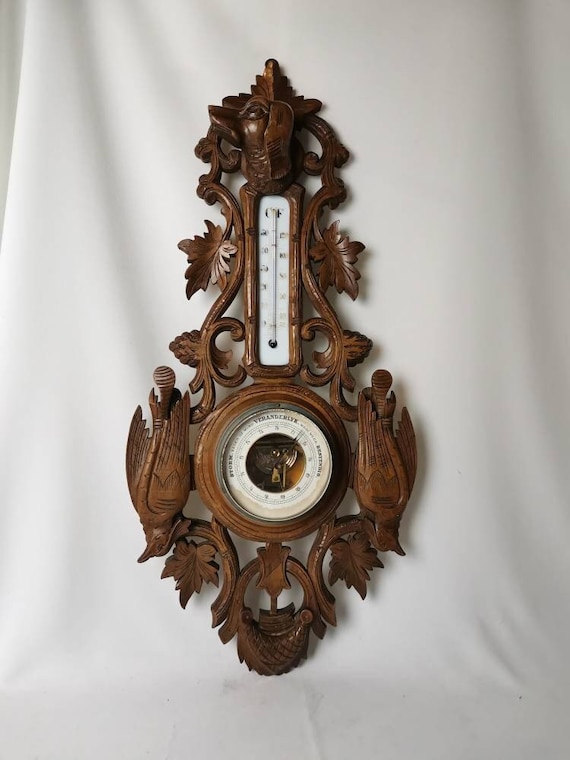The image depicts an ornate, vertical rectangular weather station with intricate, carved wooden designs. This dark, polished wood piece features elaborate carvings of leaves, half circles, and other shapes, possibly including draping branches, hummingbirds, and even a face at the top. The background is a white cloth, perhaps a drape or tablecloth, highlighting the fine details of the wooden object. At the narrow top of the structure, there's an old-fashioned thermometer with a bulb filled with liquid mercury, enclosed in a white background with numerical markings. Below this, the wood widens into a rounded, pear-shaped base, housing a barometer with a visible needle mechanism, reminiscent of vintage weather instruments that gauge atmospheric pressure. The overall craftsmanship suggests significant time and effort were invested in creating this exquisite piece.